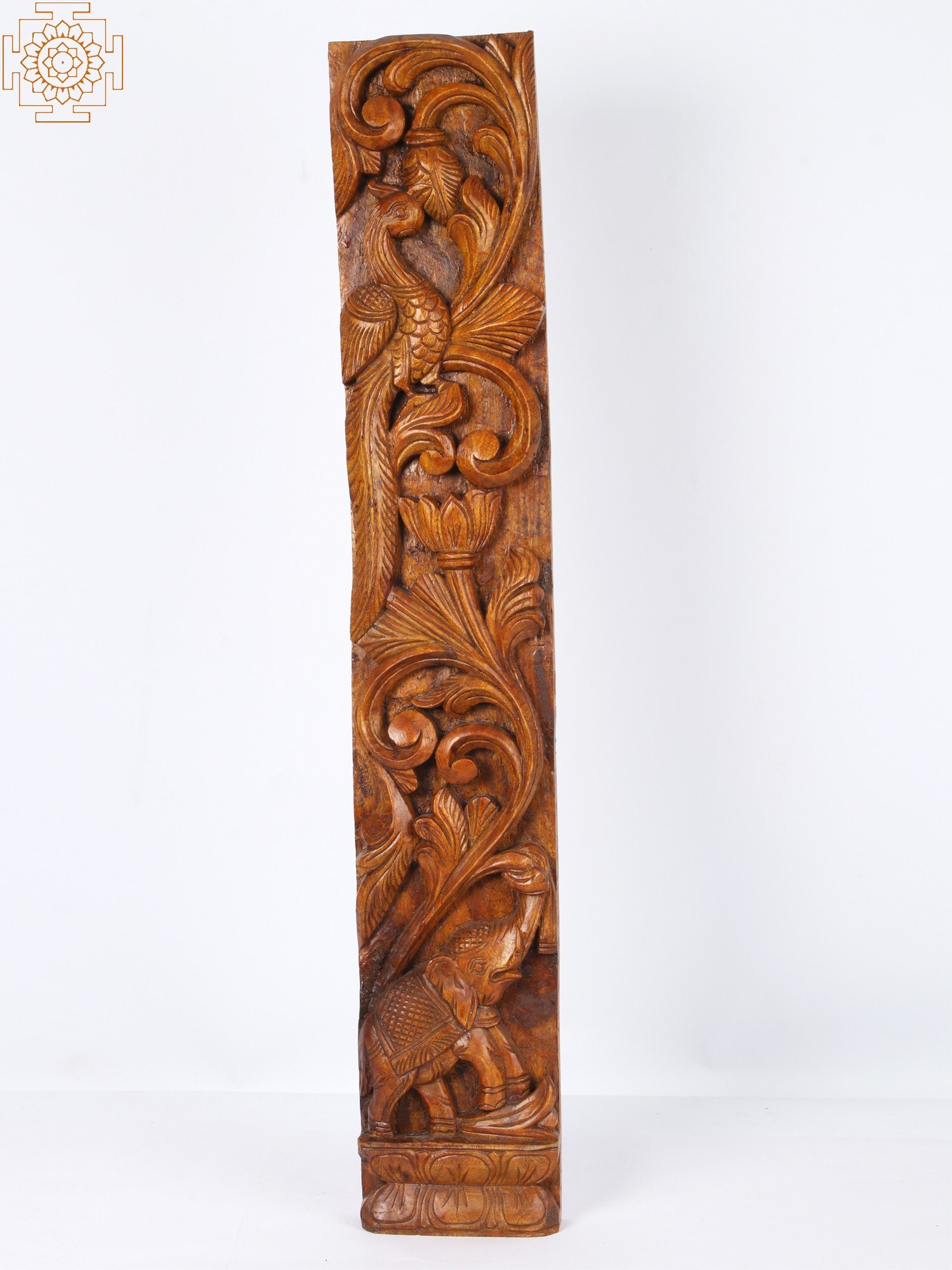This image showcases a meticulously carved wooden sculpture, lacquered in a rich walnut red tone, and set against a pristine white tabletop and background, hinting at its professional presentation, possibly for an auction or museum exhibit. The slender, elongated form of the object is reminiscent of a remote control, featuring intricate carvings that convey a narrative from base to top. At the bottom, an elephant draped in a Southeast Asian fabric is depicted, its trunk reaching up towards a flower. Above the elephant, a flower, likely a lily, connects it to a majestic peacock or phoenix with an elaborate, elongated tail. Additional carvings, including abstract decorative curves and leafy motifs, adorn the sculpture, adding layers of sophistication. Moreover, a symmetrical logo resembling a lotus flower and bordered by square and rectangular patterns is situated in the upper left corner, possibly indicating a brand or artist's insignia. The artifact exudes cultural depth and artistic finesse, making it a notable piece in any collection.